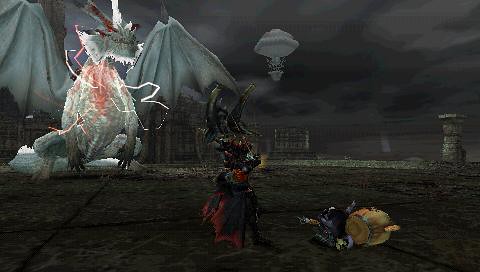This is a color photograph, likely an illustration from a video game, set against a stark black background depicting a nighttime scene. Dominating the top of the image is a dark, starless sky, allowing the other elements to stand out in vivid detail. In the middle of the scene, a silver, mushroom-shaped spaceship hovers, appearing almost ethereal against the darkness.

On the left side of the image, a striking dragon with a bright, round body takes center stage. The dragon's body features a glowing red core, contrasting against its light, translucent grey wings. The creature's head and feet are edged in white, adding a surreal glow to its form.

Centrally positioned is a character clad in a dark outfit edged with a red trim and a red top, though the details are difficult to discern due to the dim lighting of the scene. To the right of this character is a small, round yellow object, partially obscured by shadows. Adjacent to this object, and slightly protruding into the scene, is a black entity that may be machinery or another character, adding a layer of mystery to the illustration.